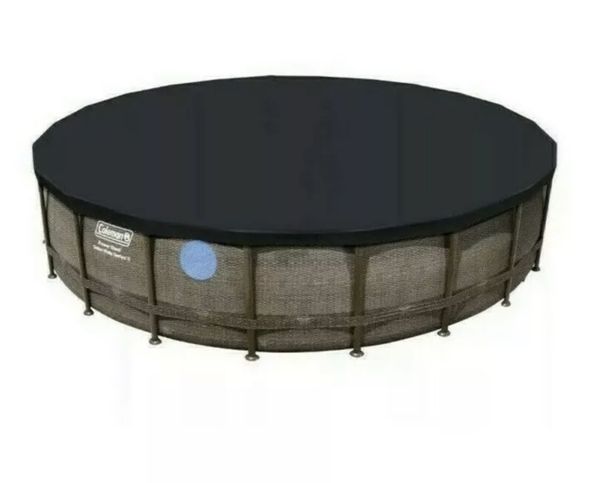The image depicts a circular trampoline with a black jumping surface on top, supported by numerous dark green or brown legs extending vertically down to the ground. A continuous dark green frame encircles the structure, holding it together. Positioned near the left side of the trampoline’s base is the brand name "Coleman" in white lettering. To the right of the logo, a light blue circular dot is prominently visible. The trampoline is situated against a white background, making its features stand out distinctly. The bottom part of the frame appears to be brown in some descriptions, giving the overall structure a robust, reinforced look.